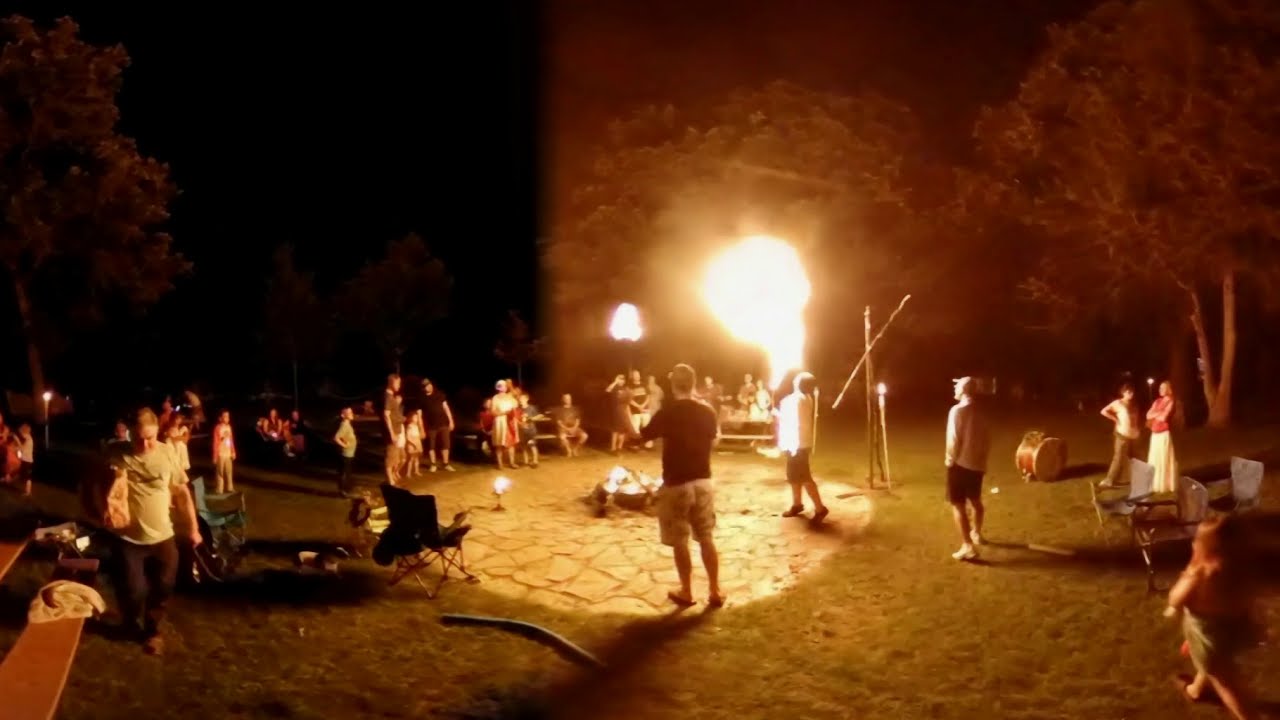The image captures a vibrant nighttime fire performance at a private outdoor gathering, likely a rave or small festival, set in a wooded area. In the center of the scene, a performer skillfully breathes vivid orange and yellow flames, captivating an audience seated on camping chairs, picnic tables, and benches arranged around a circular stone area with a campfire at its heart. The ground within the circle is stony, surrounded by lush grass. The dark sky and tiki torches add to the ambiance, while large tree canopies frame the scene, their colors altered by the flickering firelight. The atmosphere is lively and communal, with people in summer attire, possibly making s'mores and enjoying a night filled with unique, fresh performances.